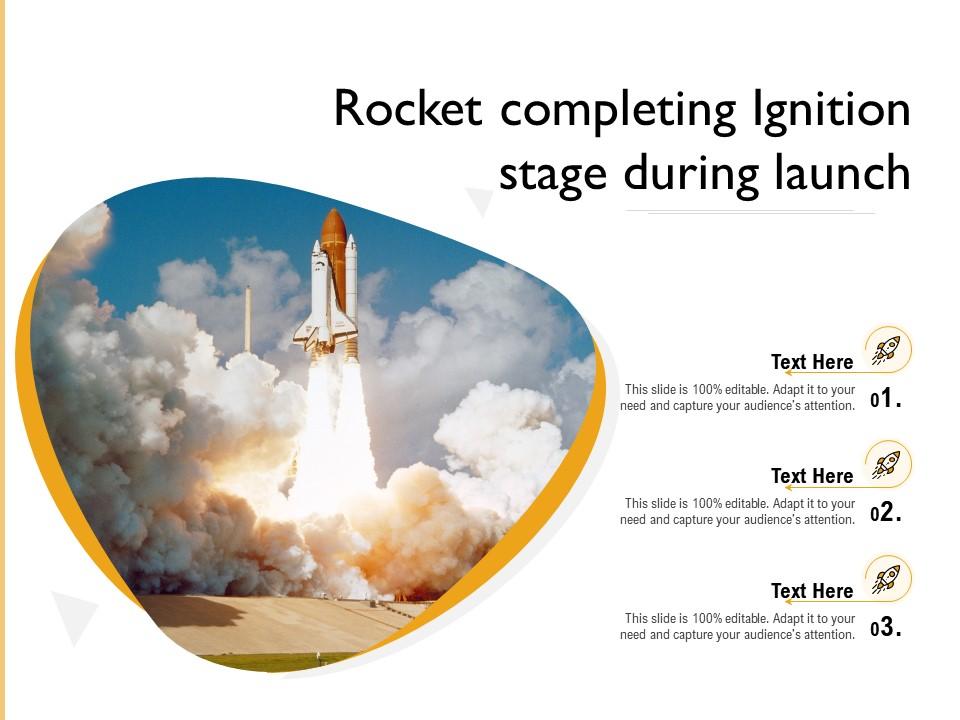The image, set within an infographic template, depicts a burnt orange, pebble-shaped photograph of a rocket launch. The rocket, distinguished by white side boosters, erupts from a concrete pad amidst a massive gray cloud of smoke, with flames visible beneath the secondary rockets. The backdrop reveals a hint of blue sky at the top and the ground below, though the thick plume of smoke dominates the center of the image. The text at the top of the infographic reads: "Rocket Completing Ignition Stage During Launch." Alongside the image, on the right, are three bullet points labeled O1, O2, and O3, each with placeholder text stating “text here” and “This slide is 100% editable. Adapt it to your need and capture your audience's attention.” A small light gray triangle points toward the photograph, and an orange line marks the left edge of the slide, suggesting a border. This setup, resembling a textbook illustration, is clearly designed as a template for presentations, inviting users to customize the content for their own use.